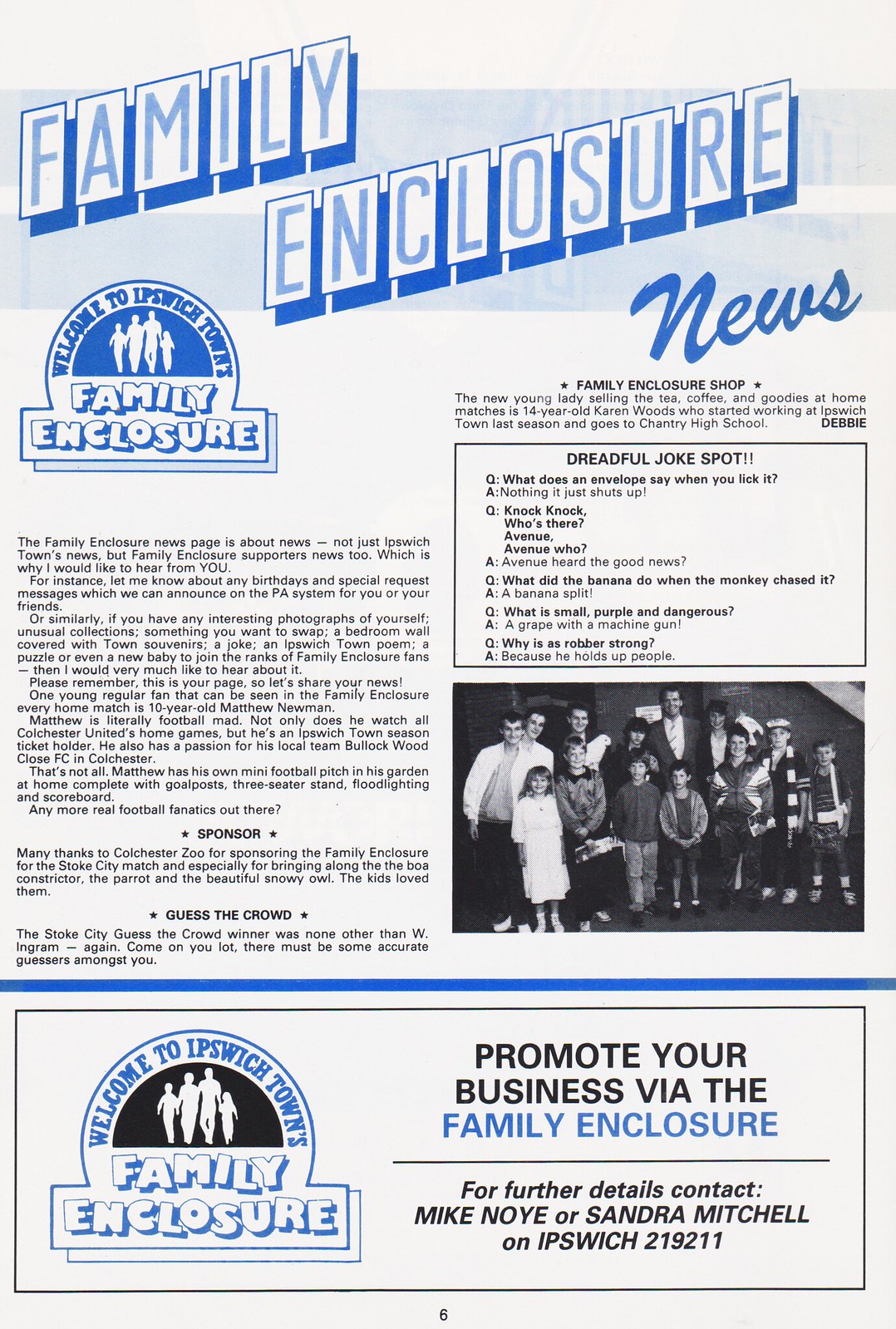The image is a scanned copy of a pamphlet or brochure, predominantly white with blue and black text. At the top, it reads "Family Enclosure News" in blue. Below that, there's a blue logo and the phrase "Welcome to Ipswich Town Family Enclosure." The central feature is a black-and-white photo showing a diverse group of about 15 men, women, and children standing together. On the right side, there is a section titled "Dreadful Joke Spot" featuring light-hearted jokes, including "What does an envelope say when you lick it? Nothing. It just shuts up." and "Why is rubber strong? Because it holds up people." At the bottom, the pamphlet encourages promoting businesses via the Family Enclosure, listing contacts as Mike Noy and Sandra Mitchell, with a phone number provided.